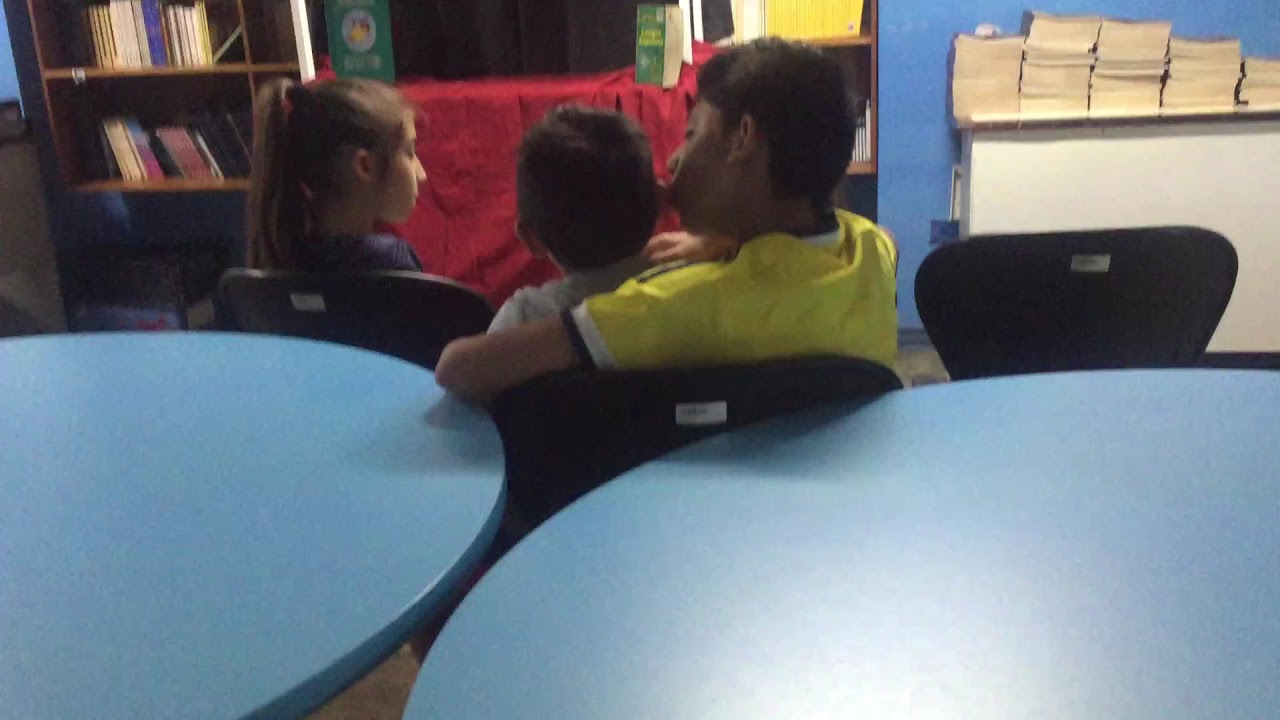This photograph depicts a scene in what appears to be a classroom or a small library with blue walls. In the foreground, there are two turquoise blue round tables with three black chairs arranged in front of them. The chairs have labels on their backs. On the leftmost chair sits a young girl with brown hair tied up in a high ponytail, wearing a blue t-shirt. She seems to have her eyes closed. 

In the middle chair, a slightly older boy is wearing a bright yellow t-shirt and has dark brown skin. He appears to be holding a younger child, who is likely just a few years old and has brown hair. The younger child is perched on his lap and is wearing a pink t-shirt. The rightmost chair is empty, as the boy has moved to the middle chair to comfort and hold the younger child.

In the background, against the blue wall, there are shelves filled with books, contributing to the cozy and educational atmosphere of the room. The children's backs are to the camera, facing the wall with the books and the tables situated behind them. The arrangement suggests a warm, familial or classroom setting, with the children gathered closely together.